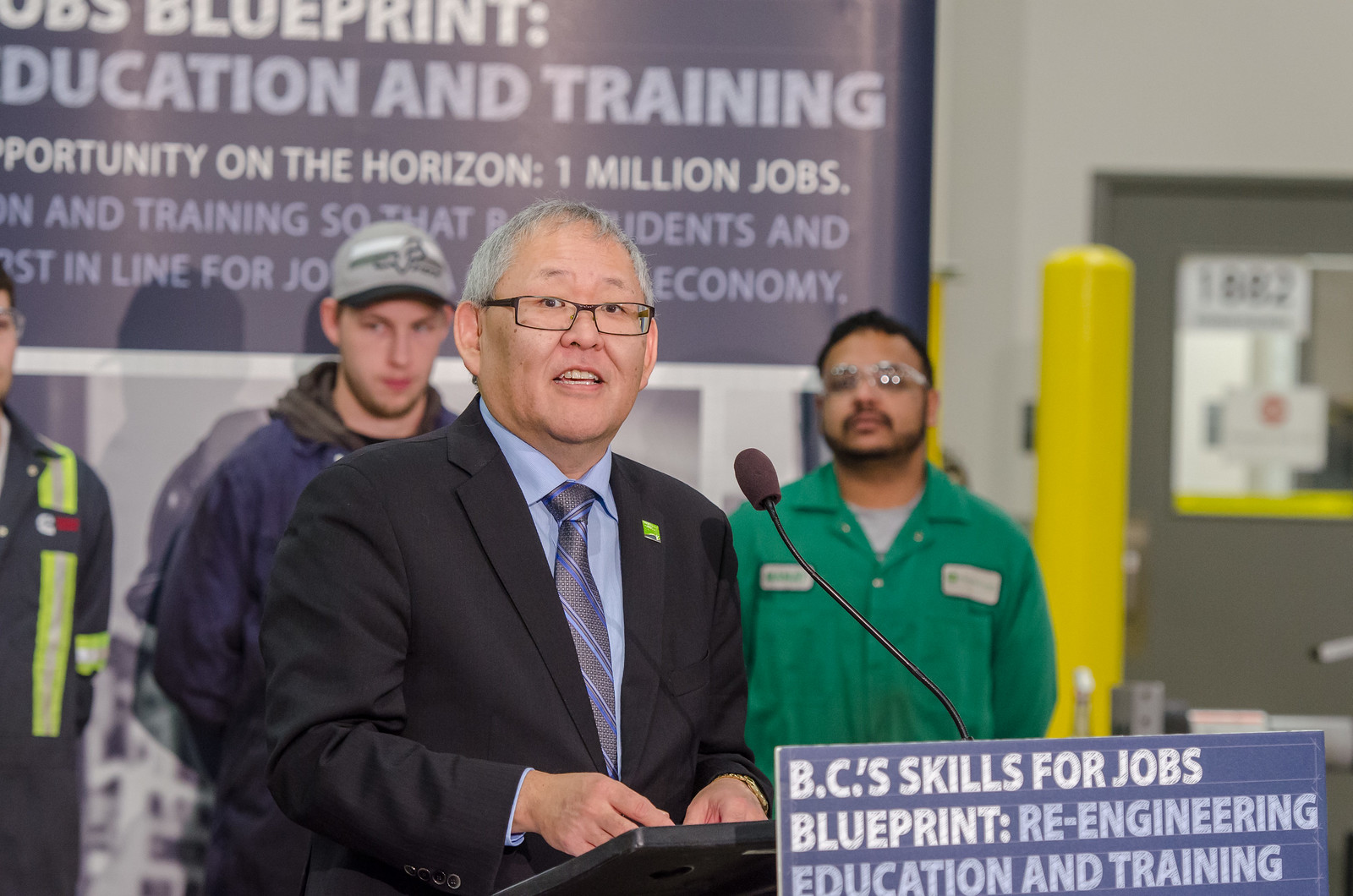The photograph, taken indoors, features an Asian man with grayish hair and black glasses giving a speech. He is positioned behind a podium adorned with a sign that reads, "BC's Skills for Jobs Blueprint" in white text, and "re-engineering education and training" in light blue. The man is dressed in a dark navy blue suit, a light blue shirt, and a grayish striped tie. His hands are gesturing in front of him as he speaks, his mouth open in mid-speech. To the right of him stands a lone microphone. 

Behind the speaker, three individuals are visible, each with their hands behind their backs. One man, likely Caucasian, wears a baseball cap and blue jacket, another to his left wears a gray work shirt with a white and fluorescent yellow safety vest. The third person, standing to the right and slightly behind the speaker, has light brown skin, possibly of Indian or Hispanic descent, and wears a green button-up collared shirt with safety goggles and what appear to be utility badges.

Suspended above the group is a larger banner echoing the sign on the podium, reading "BC's Skills for Jobs Blueprint - Education and Training," and including the additional phrase, "Opportunity on the Horizon: 1 Million Jobs." This setup suggests the event could be centered around a political or socio-economic initiative aimed at job creation or educational reform.